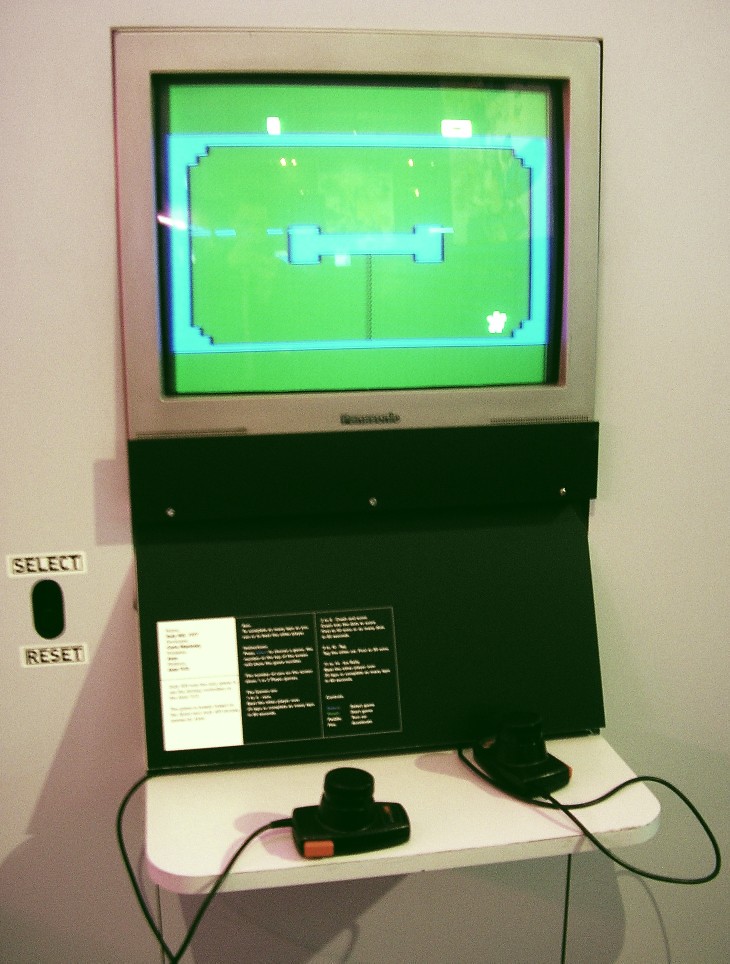The image depicts a sleek, modern computer monitor embedded into a wall, seamlessly integrated as though it's part of the structure. The screen itself is a striking lime green, accented by a blue square with a light blue outline, somewhat resembling a window with an inverted eye design centered in the blue area. Below the monitor, a black console panel hangs, featuring three distinct squares: one white and two black, each containing text.

The panel also has the word "SELECT" marked in black on its side, positioned on a white tape-like background. Centrally located on the panel is an elongated, black, oval-shaped button, and at the bottom, the word "RESET" appears, also set against a strip of white.

Directly underneath this setup rests a white shelf that supports two controllers of different designs. One of these controllers is particularly notable, featuring an orange button on its side.

The entire ensemble exudes a futuristic aesthetic while maintaining practicality and functionality.